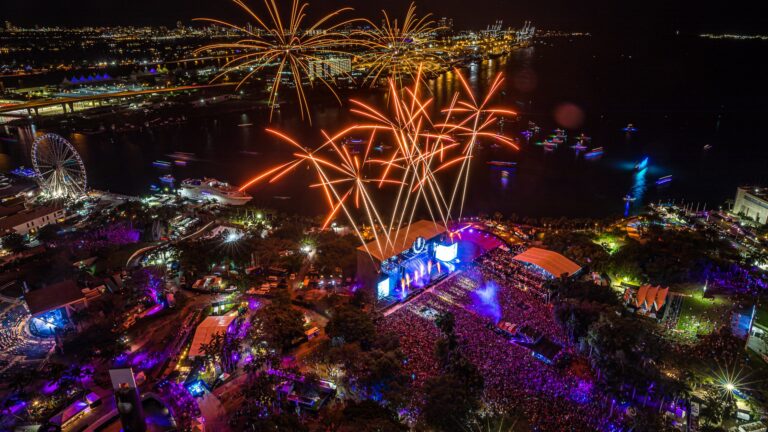The image depicts a vibrant nighttime cityscape, bustling with activity. Dominating the scene is a large, brightly lit Ferris wheel on the left side, surrounded by numerous illuminated buildings with diverse white, blue, and neon hues. The upper right corner reveals a serene body of water, dotted with various boats glowing in different colors like blue, orange, purple, and green. At the very top, and prominent throughout, fiery orange and red fireworks burst into the black sky, casting a warm glow over the scene. 

Centrally located is a crowded festival, captured as if from a high vantage point, possibly a drone or helicopter. A large stage at the heart of the crowd radiates bright blue light, washing over the attendees with a purple hue. Near the stage, an orange tent is visible, adding to the festive atmosphere. The crowd, stages, and additional events populate the left and bottom areas, while the far background showcases a striking skyline of buildings lit up with a mix of white and neon lights. Scattered greenery, including grass, trees, and bushes, adds a natural touch to the urban festival scene.